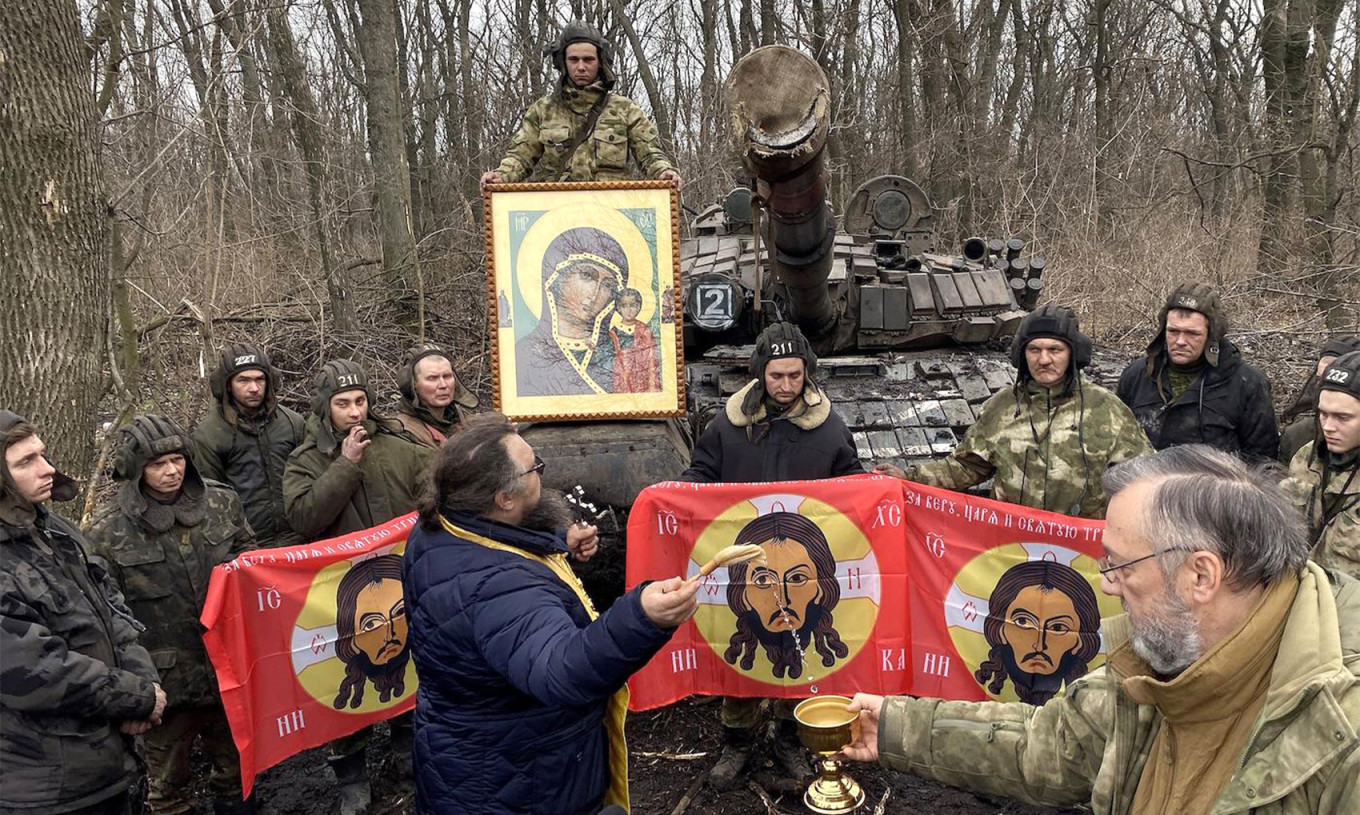In this outdoor photograph, a group of military personnel is gathered around a green tank pointed towards the camera, with a backdrop of a woodsy, somewhat barren area. Central to the composition, a soldier in green combat fatigues stands on the tank holding a large, framed painting of the Virgin Mary, depicted in an Eastern Orthodox style. Flanking the tank and positioned in front are several soldiers, most notable among them are those holding red rectangular banners featuring the face of Jesus Christ encircled in yellow, also echoing Eastern Orthodox iconography.

In the front center of the group, two men stand out. The man on the left wears a green camouflage jacket and holds a golden goblet, while the man to his right, dressed in a blue winter coat, dips a brush into the goblet, which is dripping water as he raises it in the air, presumably performing a blessing. This man also clutches a gold cross partially hidden behind his full beard. All the soldiers appear to be wearing padded tank helmets, emphasizing their combat readiness. The scene captures a blend of military and religious imagery, highlighting a moment of spiritual observance amid a martial setting.